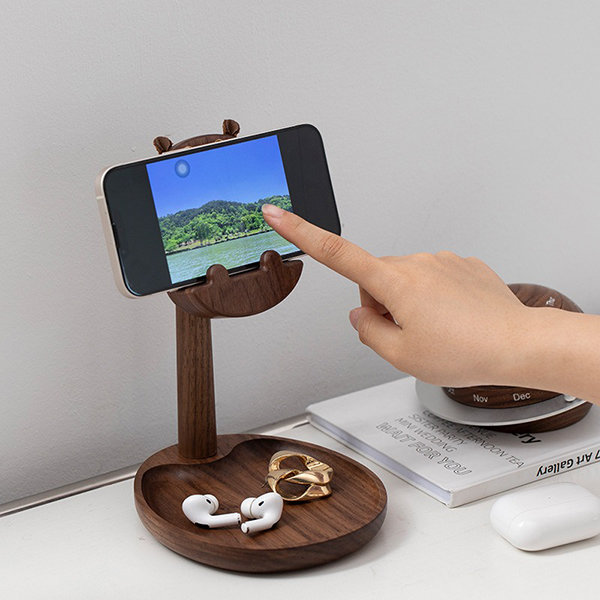The image depicts a lightly off-white countertop against a matching off-white wall. The separation line between the wall and the counter ranges from about 20% up on the left to around 40% up on the right. Positioned on the left-hand side of the counter is a multi-functional wooden stand with a round, bowl-like base. This base serves as a tray and contains a couple of earrings, a pair of wireless ear pods, and their case. Attached to the stand is a pole supporting a circular cell phone holder, which currently cradles a white iPhone positioned horizontally. The iPhone displays a scenic photo featuring a beach with water, trees, and sky. A Caucasian hand is seen touching the right side of the screen. Adjacent to the wooden stand, there lies an art gallery book, partially visible with various objects resting on it.